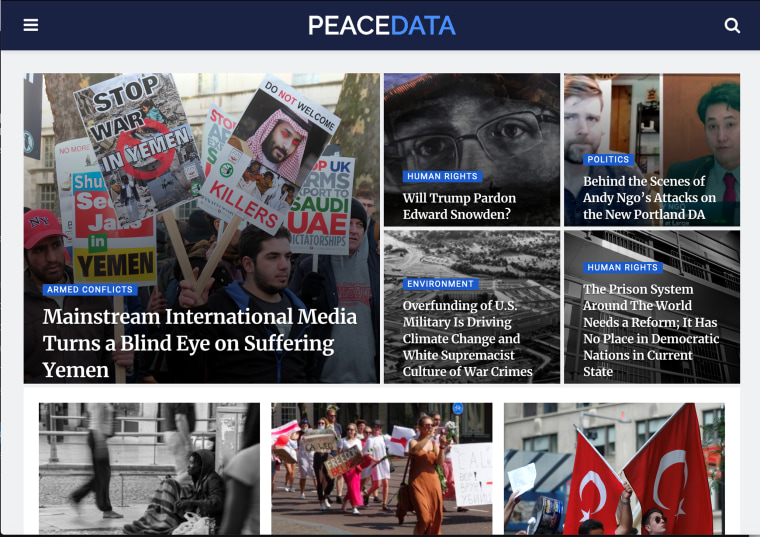This image is a detailed screenshot from a website named PeaceData, where "Peace" is written in white and "Data" in light blue text, both centrally positioned on a navy blue banner at the top of the page. The banner also features a hamburger menu in the upper left corner and a search icon in the upper right corner. The main body of the screenshot displays several clickable content boxes categorized under different banners with corresponding article titles. 

The leftmost box, labeled "Armed Conflicts" in white text on a blue banner, features an article titled "Mainstream International Media Turns a Blind Eye on Suffering in Yemen." Other articles shown include topics like "Human Rights: Will Trump Pardon Edward Snowden?" and "Politics: Behind the Scenes of Andy Ngo's Attacks on the New Portland DA." Additional content covers "Environment: Overfunding of the US Military to Drive Climate Change and the White Supremacist Culture of War Crimes," and "Human Rights: The Prison System Around the World Needs Reform - It Has No Place in Democratic Nations in its Current State." This website appears to offer a critical and in-depth examination of various pressing global issues.